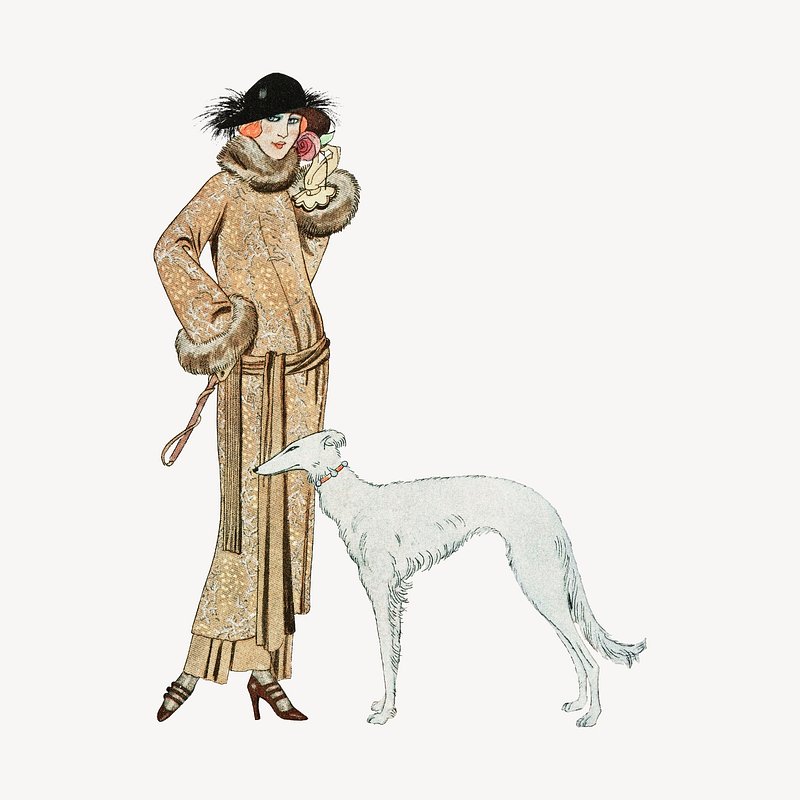An illustration, evocative of the Art Nouveau or Art Deco style of the 1920s, features a woman and her slender white greyhound. The woman, with her short orange hair and striking makeup of red lips, blush, and blue eye shadow, stands poised in a long, fur-lined coat that extends to her ankles. The beige-brown coat is adorned with fur around the collar, cuffs, and the drooped waist, accentuated by a belt-like scarf. She wears a black wide-brimmed hat embellished with feathers and puffs of fur, and her ensemble is completed with red high-heeled shoes and orange earrings. In one hand, she elegantly grasps a baton and a rose. The sleek greyhound, standing attentively in front of her, showcases a graceful, slender form typical of racing breeds, with a shaggy tail and a pearl collar around its neck. This detailed depiction captures both the elegance and the period-specific charm of the subjects.